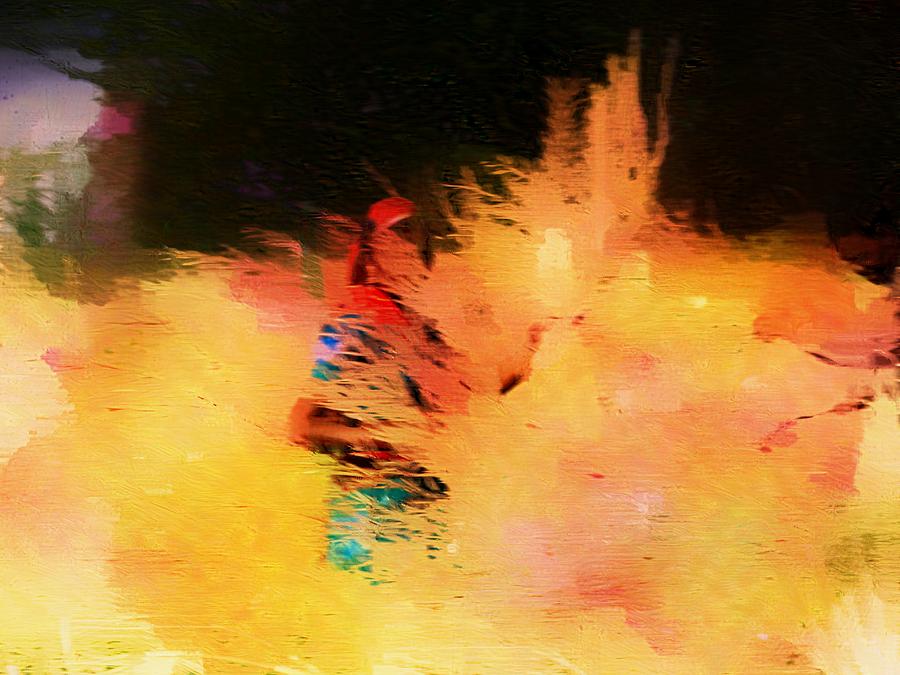The image showcases an abstract painting rendered in a landscape orientation. It features a dynamic interplay of colors and textures, predominantly characterized by splotches of light in various hues of yellow surrounded by rich reds, evoking the chaotic intensity of fire. Toward the center-right, there's a sense of movement angling upward to the top right, suggesting energy and motion. In the foreground, the abstract shapes coalesce into a discernible figure—a woman of darker skin wearing a red headscarf and an indistinct dress in tones of blue, white, and green. Her form blends fluidly into the surrounding colors, as if standing amidst a vibrant, roaring landscape. The painting exhibits depth through a contrasting dark or shadowy section at the front center, transitioning into pitch-black at the top, except for a softer light pink or purple area with green, perhaps hinting at foliage. The overall palette includes striking warm colors—reds, yellows, and oranges at the bottom—which merge with cooler blues and greens towards the top. This vibrant contrast of warm and cool tones, accented by patches of purple, imbues the painting with a powerful and immersive depth, embodying the essence of abstract art's emotive and ambiguous nature.